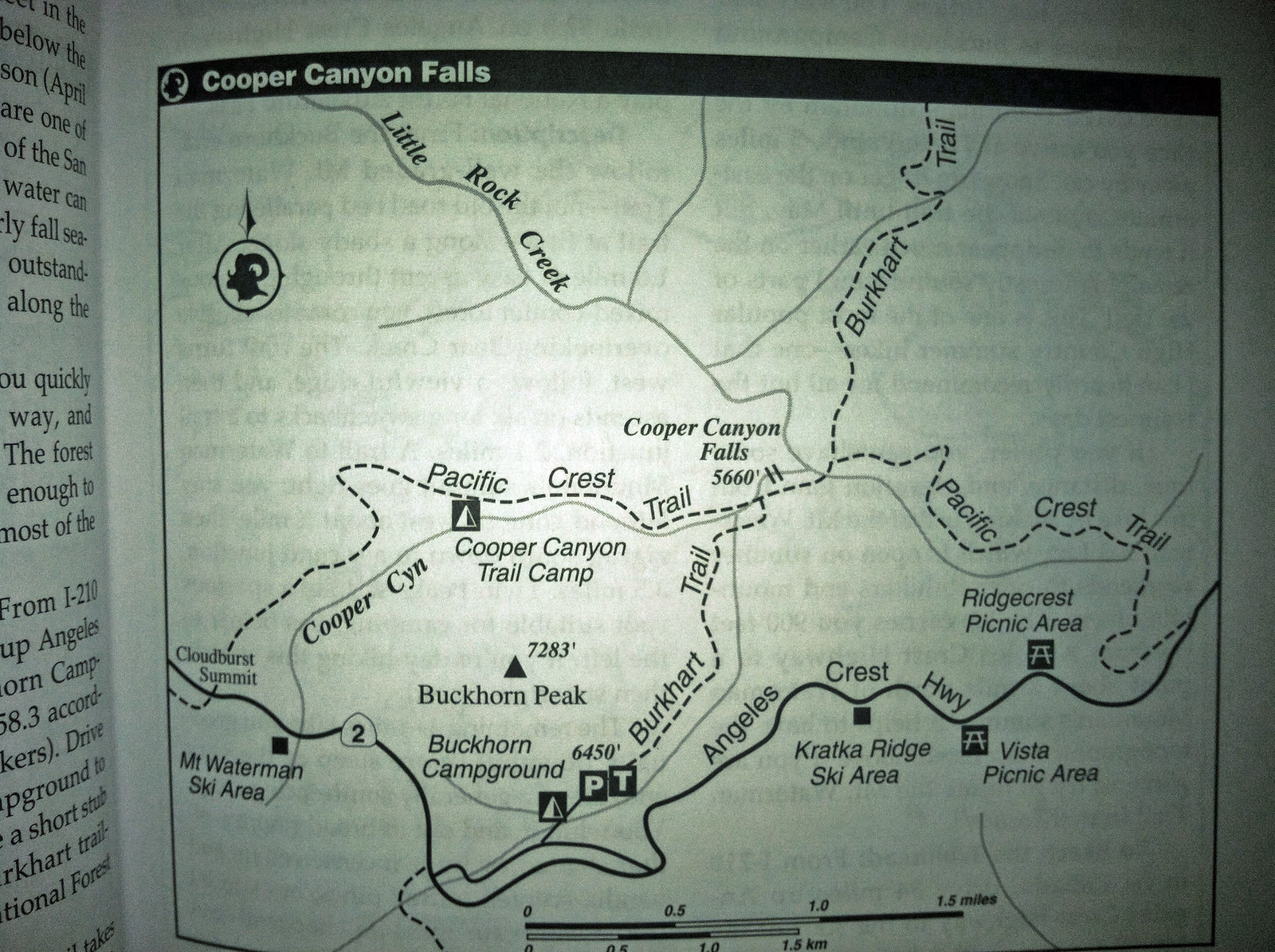The image is a black-and-white photo of a page from a book or pamphlet detailing a hiking map titled "Cooper Canyon Falls." The page is on the right side of an open book and has a prominent black header with the title "Cooper Canyon Falls" in bold white text. The page features a rectangular map showing various trails and geographical features including the Pacific Crest Trail, Burkhart Trail, Little Rock Creek, and the Angeles Crest Highway. Additionally, Buckhorn Peak is marked on the map. There is a black compass at the bottom, emphasizing the north direction, and a scale in both miles and kilometers at the bottom of the map. The left edge of the page contains partial text from an adjacent page, visible only as fragmented lines of text.